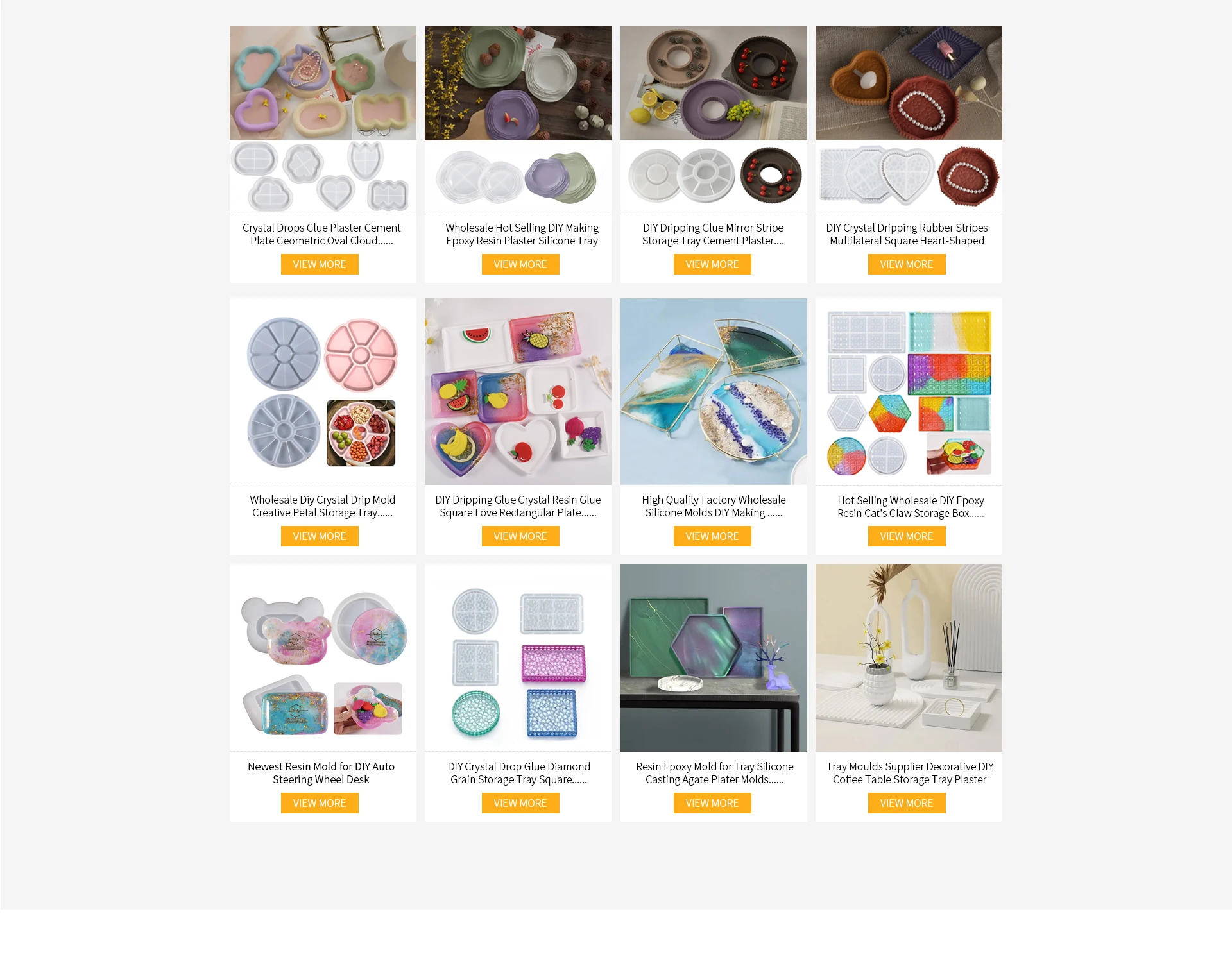In the image, we're presented with a selection of assorted kitchen and crafting utensils showcased on an online retailer's website. The display features 12 distinct items, each accompanied by an orange or yellow "View More" button for further details. The items available for purchase include various materials and DIY tools such as crystal drops, glue, plaster, cement, and silicone trays. Specific products highlighted are a geometric oval cloud, hot-selling epoxy resin molds, storage trays, and multilateral square and heart-shaped rubber strips, all designed for creating personalized household items. These tools and materials come in a vibrant array of colors, catering to diverse crafting needs and preferences.